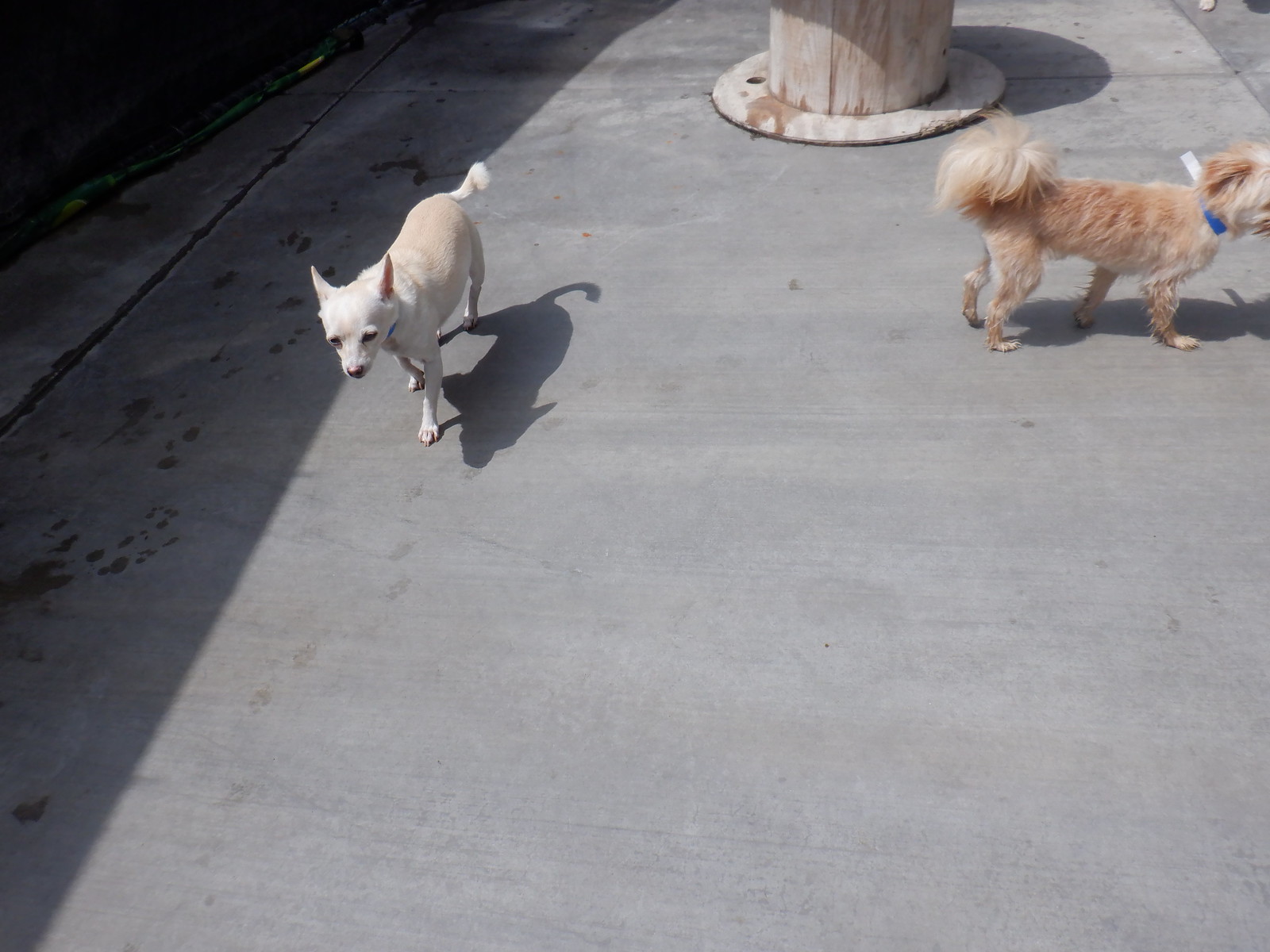In this outdoor concrete setting, likely a patio or city sidewalk, two small dogs are strolling in the sunlight. The scene features part of a brown circular table and their pronounced shadows indicating the bright conditions. On the left, a white, short-haired dog with pointy ears and a curled short tail is walking towards the viewer, wearing a blue collar. To the right, a cream-colored dog with hints of rust in its longer fur, also adorned with a blue collar, is looking sideways with its bushy tail held high. Both dogs, each weighing around 7-8 pounds, appear to be content as they navigate the concrete, although the harsh surface contrasts with their need for softer ground.